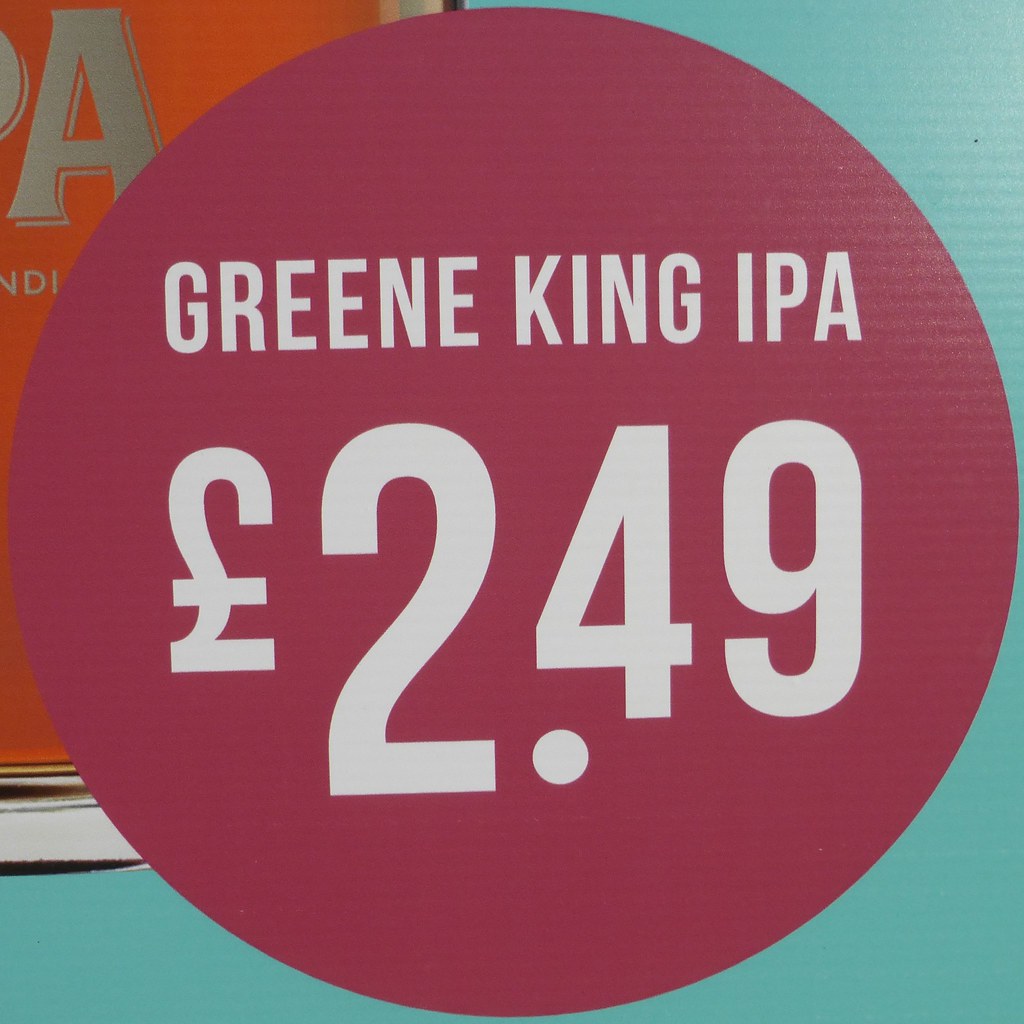The image features a square label with a sky-blue background extending across the top right and lower left. Dominating the center of the label is a large, solid burgundy circle that nearly touches the edges of the square. Inside this circle, the text "Greene King IPA" is prominently displayed in white, with "Greene" spelling out the traditional English greeting with an extra 'e'. Beneath the brand name, the price "£2.49" is also printed in white, signifying the cost of the beer in British pounds. The top and right sides of the circle are flanked by a cyan background, while in the upper left, a portion of a beer glass is visible alongside a cut-off letter "A." Additionally, there is an orange background at the bottom left adorned with partial silver lettering that appears to spell out "ANDI". The detailed design elements and color contrasts surrounding the focal circle together create a vibrant backdrop for the label.